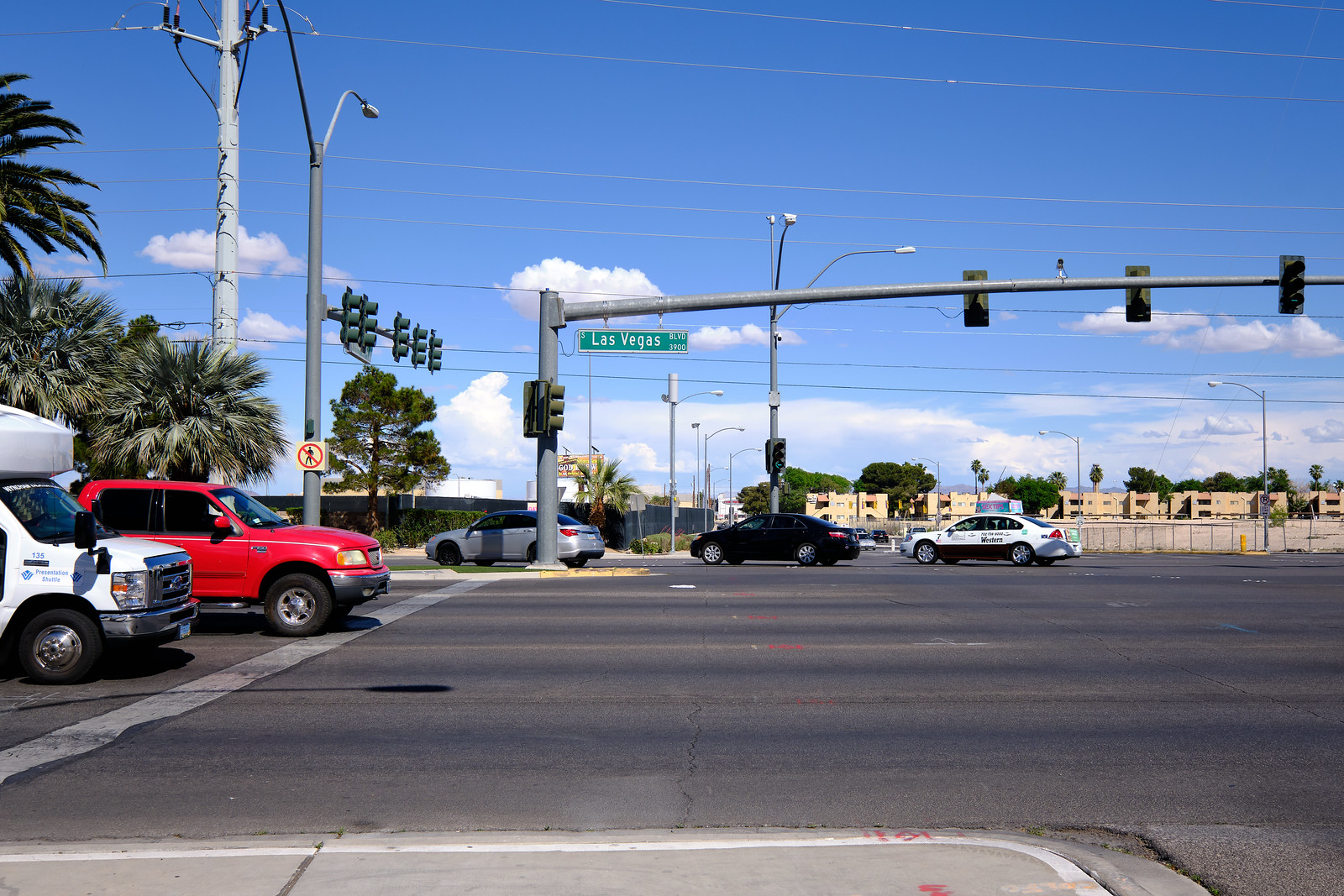This photograph captures a bustling highway, likely in Las Vegas, as suggested by the prominent green road sign in the top-middle of the image that reads "Las Vegas." The foreground features a paved multi-lane road, approximately three or four lanes wide, stretching from the middle left to the right side of the frame. A distinct white stop line marks where vehicles halt for the traffic light. 

On the road, a red car is heading to the right, followed closely by a white truck on its right side. Towards the middle right, a white car with visible writing on its body is traveling in the opposite direction, leftward, closely trailed by a black car and a gray one ahead of it.

The upper portion of the scene is dominated by an array of traffic lights suspended on poles, spanning from the top right to the left side of the photograph, along with additional poles indicating directions of different lanes. Numerous electric lines crisscross above, contributing to the urban atmosphere.

In the background, several buildings, possibly apartment complexes made of brown brick or stone, stand against a backdrop of a bright blue sky adorned with fluffy white clouds, completing this lively urban snapshot.